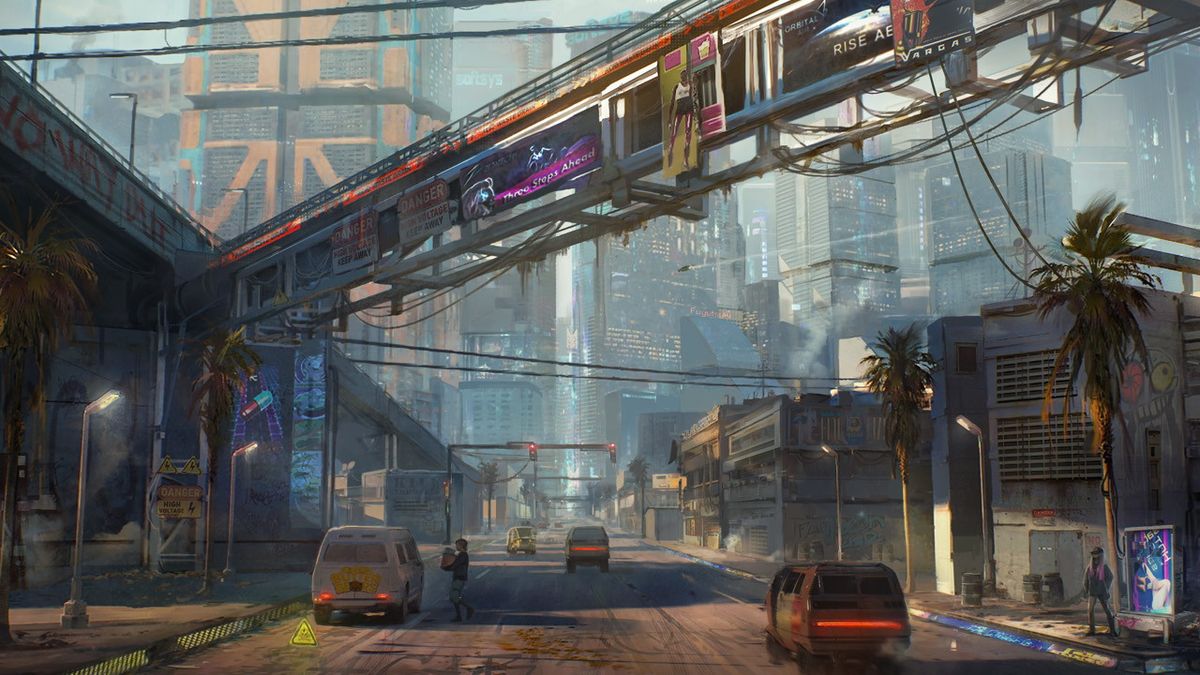This is a digitally generated image of a sprawling, futuristic cityscape, possibly inspired by a cyberpunk setting. The city is depicted as a blend of decaying urban sprawl and towering high-tech skyscrapers that stretch into a smog-filled sky. In the foreground, we see a wide street lined with small, run-down buildings and shops, cluttered with graffiti, including images of robots. Palm trees dot the sidewalks, where a few pedestrians can be seen, including one near a sign suggesting an adult entertainment venue.

The road is bustling with a mixture of decrepit cars and more advanced hovercrafts, hinting at a blend of old and new technologies. Above the street, an overpass adorned with signs reading "Danger: High Voltage" and similar warnings spans the scene. Electrical poles and wires hang haphazardly, contributing to the disarray. The overpass might also function as train tracks, adding to the layered complexity of the city's infrastructure.

In the distance, the city transitions into a more affluent area, with colossal buildings rising majestically, suggesting a stark contrast between different parts of the city. The sunlight illuminates the scene, highlighting both the grime of the rundown areas and the gleam of the distant skyscrapers. The overall atmosphere is one of a once-majestic metropolis now swathed in neglect and decay, yet still bustling with life and activity.